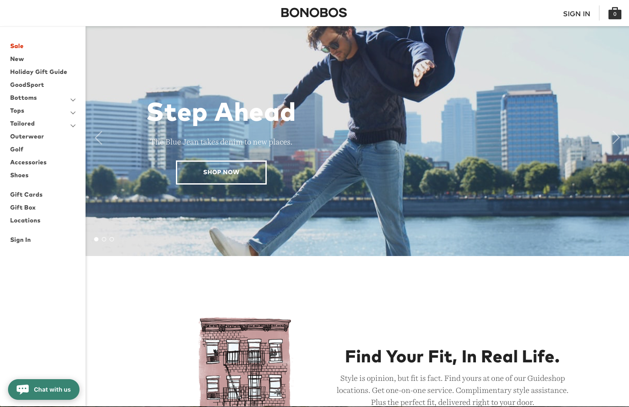This website features a clean, white background with a minimalist design that's both stylish and user-friendly. Centered at the top in bold, uppercase letters is the brand name "BONOBOS." To the right, you find options to "Sign In," and a black shopping bag icon with a zero, indicating an empty cart.

Down the left side, a vertical banner provides easy navigation through the site’s categories. It starts with "Sale" in an eye-catching orangish-red color, followed by "New," "Holiday Gift Guide," and the uniquely stylized "Good Sport" with capitalized initials. Further categories include "Bottoms," "Tops," and "Tailored," each equipped with convenient drop-down menus for more specific options. You also see straightforward sections: "Outerwear," "Golf," "Accessories," "Shoes." Additional useful links ensure you don’t miss essentials like "Gift Cards," "Gift Box," "Locations," and another "Sign In" link, designed for seamless user experience.

At the bottom of the left banner is a green tab labeled “Chat with Us” in white text, offering easy access to live customer support. 

Central to the homepage is an inviting image depicting an outdoor scene with office buildings, some trees, and a waterway against a clear sky. Below the image, a tagline in bold text reads, "Find Your Fit in Real Life," encouraging users to explore further. This webpage is thoughtfully designed to be both visually appealing and functionally efficient.